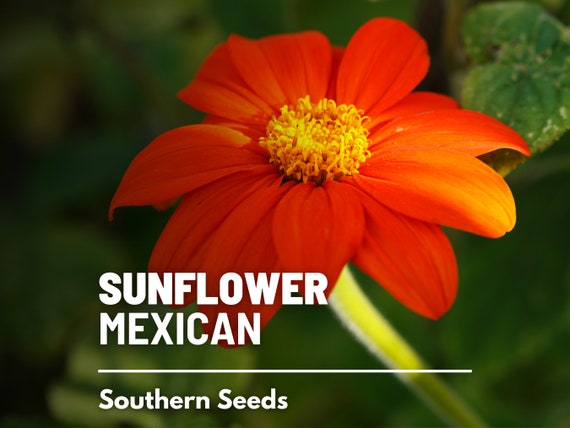This close-up photograph, possibly the cover of a seed packet or an advertisement for seeds, features a prominently displayed flower labeled in white font as "Sunflower Mexican," underlined, with "Southern Seeds" written below the line. The flower, reminiscent of a marigold or daisy, boasts deep orange-red petals surrounding a yellow center with wiry-looking yellow filaments. The stem is a light spring green, extending downward from the vibrant bloom. The background consists of blurred-out greenery and leaves, creating a soft, olive-forest green canvas that contrasts sharply with the detailed, sharply outlined flower in the foreground.